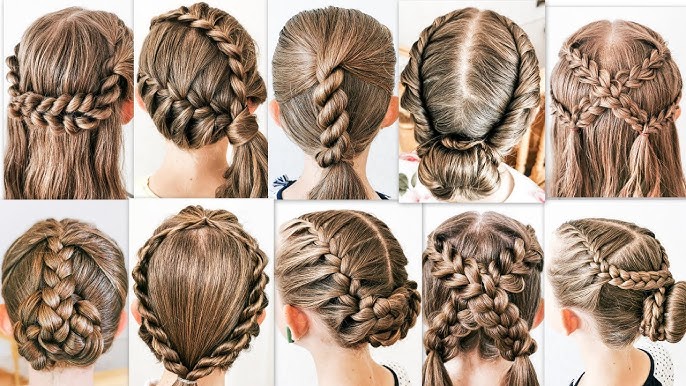This image features a detailed sequence of 10 photographs arranged in a 2x5 grid, each showcasing the back of a young woman's head with long, light brunette hair, possibly the same woman in each shot. Each photo presents a unique braided hairstyle, illustrating the diverse methods of braiding hair. The styles range from a straight-across braid at the nape to intricate braids sweeping over the top of the head. Traditional straight-down braids appear alongside more creative styles—including crossing braids, looping designs, and buns. This compilation could easily serve as a reference in a hair salon, book, or website, providing various inspirations for braiding and arranging hair in imaginative and stylish ways.